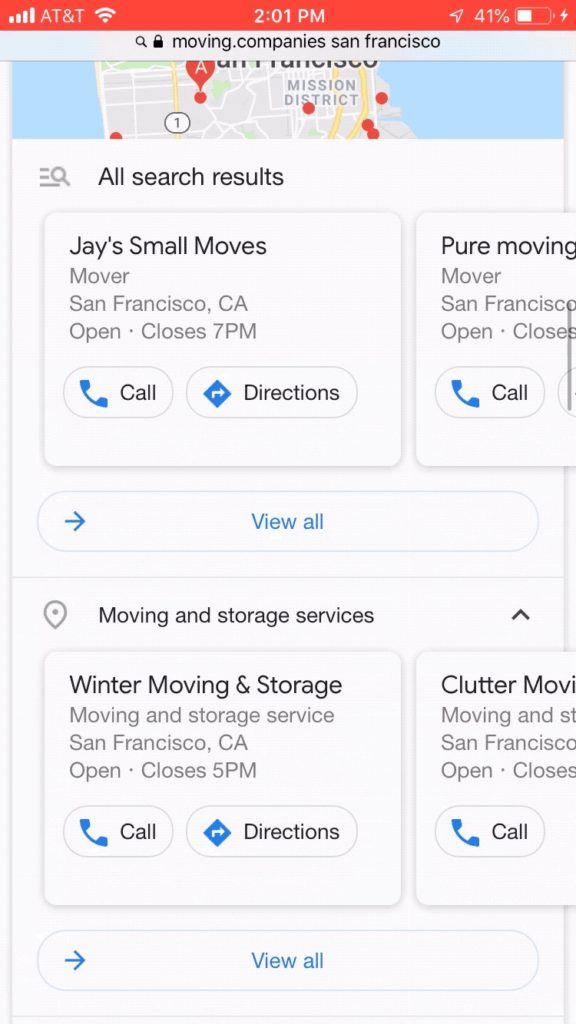This is a detailed screenshot of a search conducted on an AT&T phone. At the top, a red notification bar is prominently displayed, showing the time, 2:01 p.m., in white text. Below the notification bar, there is a partially visible map with several red dots marking various locations. The search query executed is "moving company San Francisco," followed by several results under the "All" search category.

The first result is displayed in a white box, with "J Small Moves" prominently listed as a mover located in San Francisco, California. It specifies that the business is open and closes at 7 p.m. Below this information, there are clickable options for "Call" and "Directions."

The second result, positioned to the right in another white box, is for "Pure Moving," another moving service in San Francisco. The description includes the open and close times, but the latter part is cut off and not fully legible.

At the bottom of the screenshot, an arrow icon is situated in the middle of the screen with the text "View All" beneath it, inviting the user to explore more search results. Directly below this, two more service options are presented. On the left side, "Winter Moving and Storage," identified as a moving and storage service in San Francisco, California, is listed. Adjacent to this, on the right side, is "Clutter Moving," another moving service option.